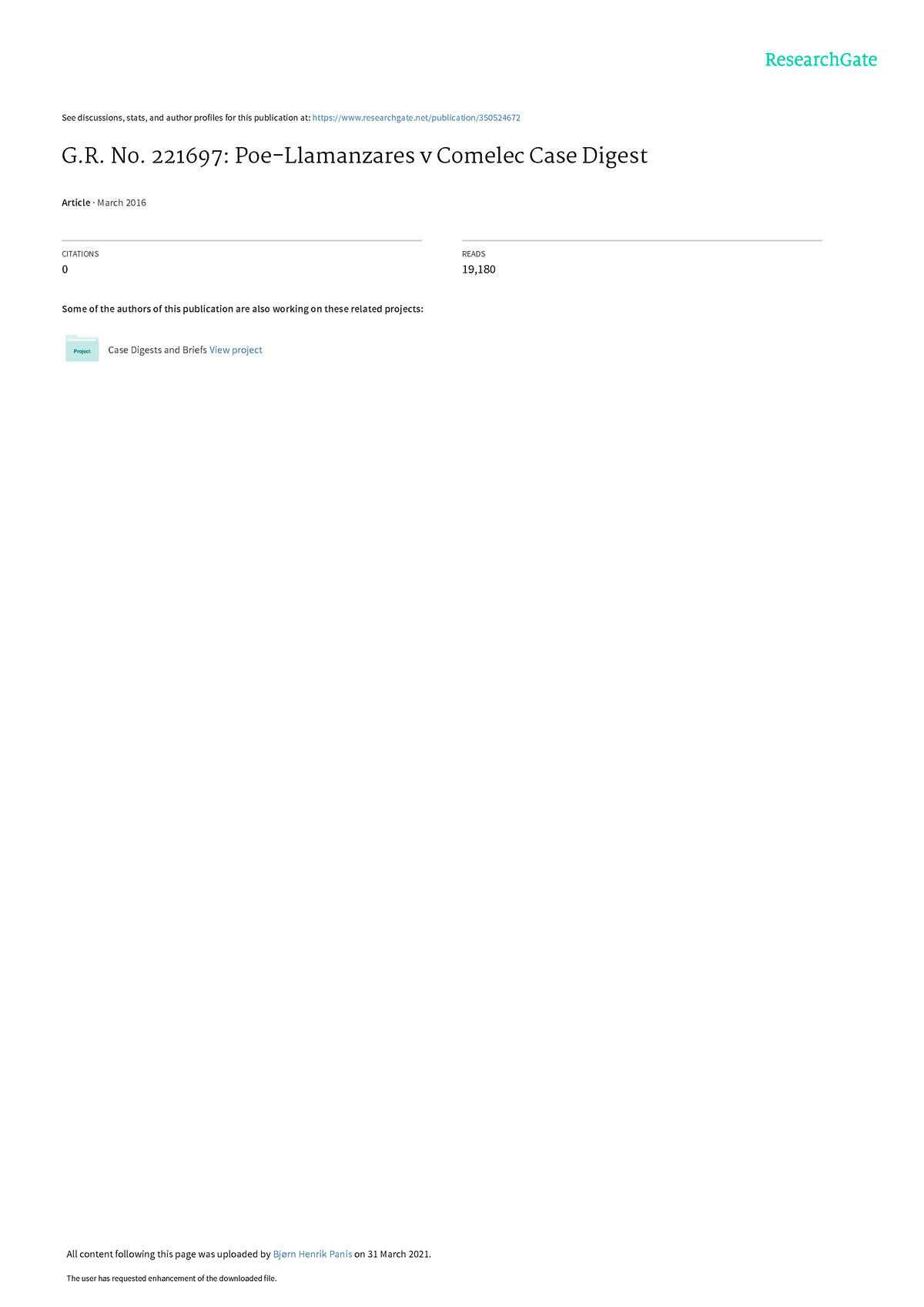A sparsely populated ResearchGate page appears, featuring a predominantly white background. In the top right corner, the "ResearchGate" logo is visible in greenish text, presented as a single word. Below, the page provides a link to "See discussions, stats, and author profiles for this publication at ResearchGate." 

The main content includes technical details such as "GR number 221697" and "Poe-Lamanzaris versus Komelec Case and Digest." The page notes that this article, published in March 2016, has zero citations and 19,000 reads. There is a mention that some authors involved in this publication are also working on related projects, suggesting that this might be of interest to professionals like lawyers, attorneys, or judges in the field.

Scrolling to the very bottom of the otherwise empty page, a note reveals that all content was uploaded by Bjorn [last name unspecified] on March 21st, 2021.